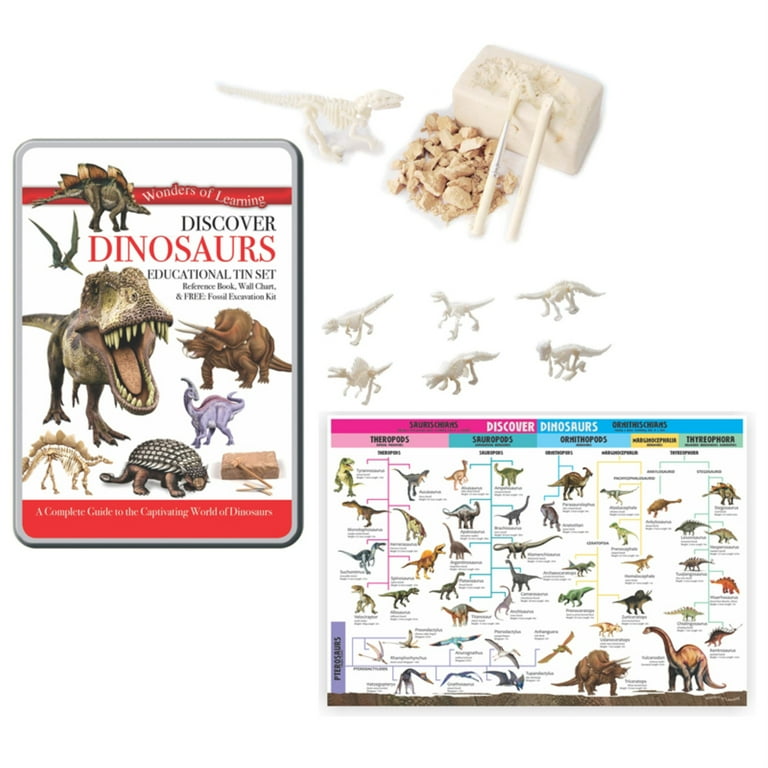This image features a detailed dinosaur activity kit for children, designed as an educational tool. The main product is a sturdy tin box, prominently displayed on the left, showcasing vibrant shades of red, pink, lighter pinks, light blue, light green, blue, black, white, gray, and beige. The tin's borders are gray, and its surface is adorned with various dinosaur illustrations. The background is a clean, white color, enhancing visibility.

The text on the tin reads "Wonders of Learning: Discover Dinosaurs," accompanied by promises of educational content and interactive fun. Within the tin, customers will find a comprehensive set that includes a reference book, wall chart, and a free fossil examination kit, making it an all-in-one resource for young paleontologists.

To the right of the tin box, in the top middle of the image, the contents of the kit are laid out clearly. There are five small, white miniature dinosaur figures, white-colored bricks, a paintbrush, and some brown stones. Just below these items, a detailed diagram showcases a classification chart of various dinosaurs.

The bottom right corner features a vibrant flowchart divided into color-coded sections, each representing different dinosaur groups such as Theropods, Ornithopods, and others. Each section is identified by its unique color—dark green, pink, blue, red, light green, and purple—with detailed descriptions and colorful flowcharts that outline various dinosaur types within each group. This engaging layout not only beautifies the presentation but also enhances the educational value, helping children easily grasp complex information.

In summary, this dinosaur activity kit is a comprehensive educational tencent combining vibrant visuals and informative content designed to captivate and educate young dinosaur enthusiasts.